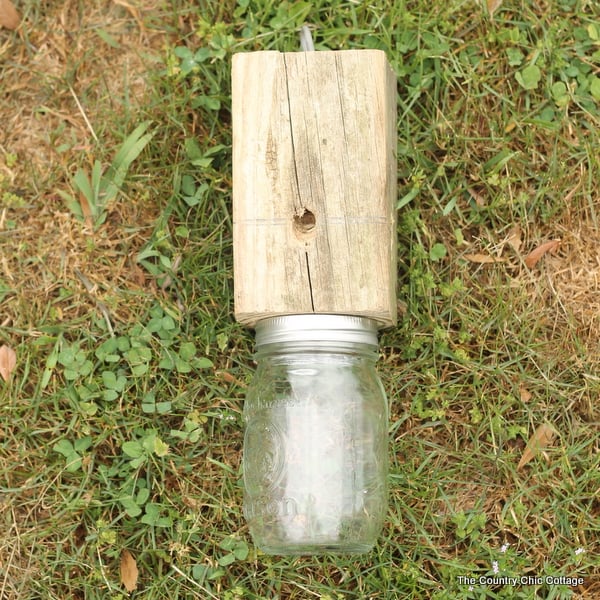In this image, we see a clear, empty mason jar with a faint yellow, silver lid attached to a rectangular wooden block at the top. There's a diagonal break in the wood, with something silver, like a screw, sticking out from the top. The entire scene is viewed from a top-down perspective, captured under bright daylight, causing a glare on the glass jar, indicating a light source from above. The jar and wooden block lie on a mixed patch of green grass interspersed with patches of yellow, hay-like grass, and brown leaves. Small clovers are visible in the bottom left and top right corners, adding detail to the lawn. At the bottom right corner, the image features the text "The Country Chic Cottage" in small white letters.